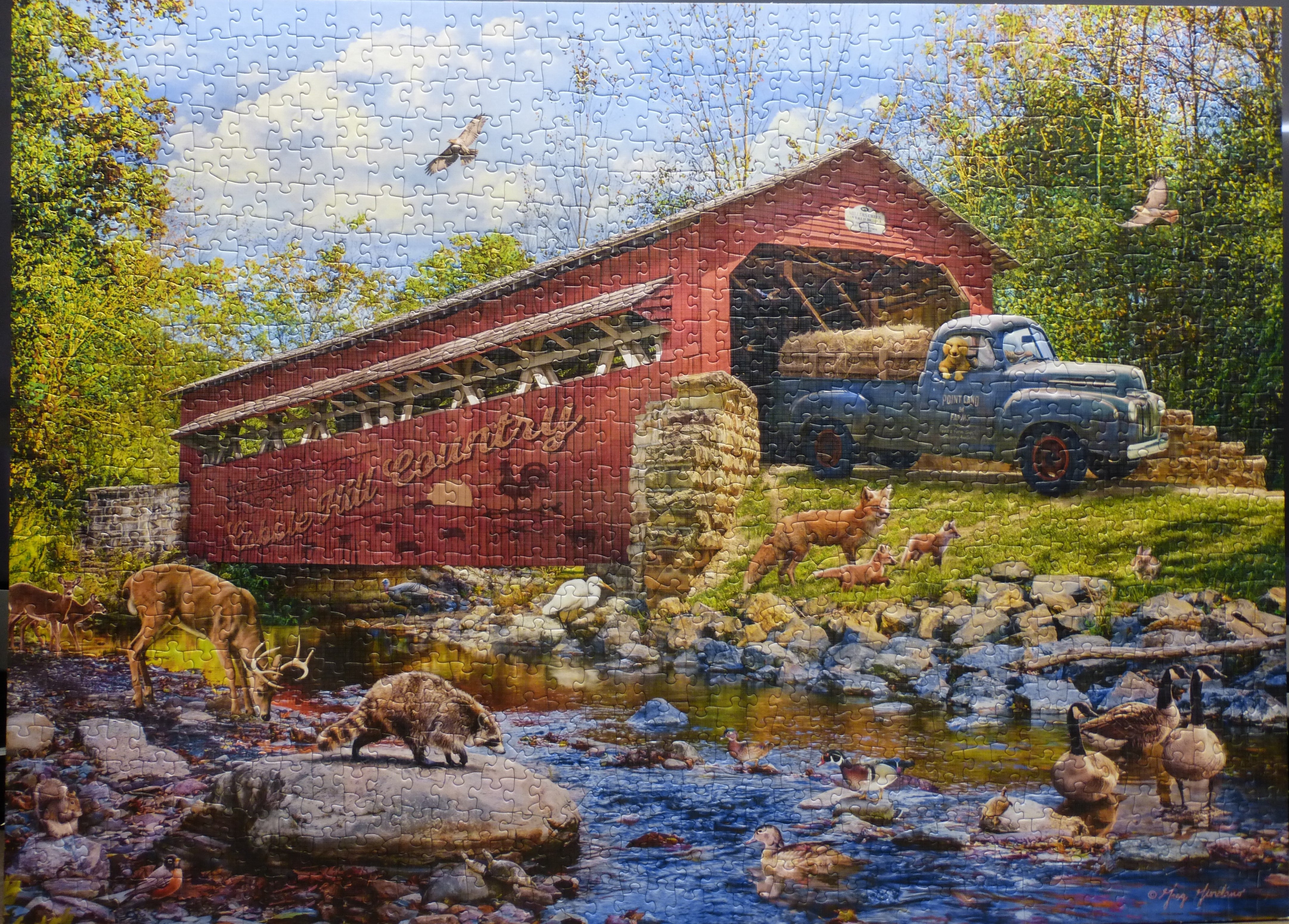This horizontal, rectangular image depicts a detailed rural scene, seemingly a painting or a photograph of a puzzle. At the center is a striking red covered bridge with louvers on its sides and a stone base visible from this angle. A vintage blue pickup truck, laden with hay and featuring a dog leaning out the window, emerges from the bridge. Inscribed on the bridge's side is "Cable Hill Country" in beige text. The scene is enveloped in greenery, with lush trees flanking either side, their green leaves backed by a light blue sky dotted with fluffy white clouds.

In the foreground, a serene stream flows, bordered by rocks and alive with various wildlife. On one bank of the stream, a deer drinks from the water, while nearby, a raccoon stands atop a large gray rock. Also within the stream are ducks and Canadian geese. A gentle green hill descends to the water's edge, home to a mother fox and her two playful cubs.

The panoramic background is rich with further details—a hawk circles in the blue sky, adding to the scene's tranquility and natural charm. This image vividly captures the essence of rural life, blending nature, wildlife, and rustic architecture into a harmonious and idyllic vista.